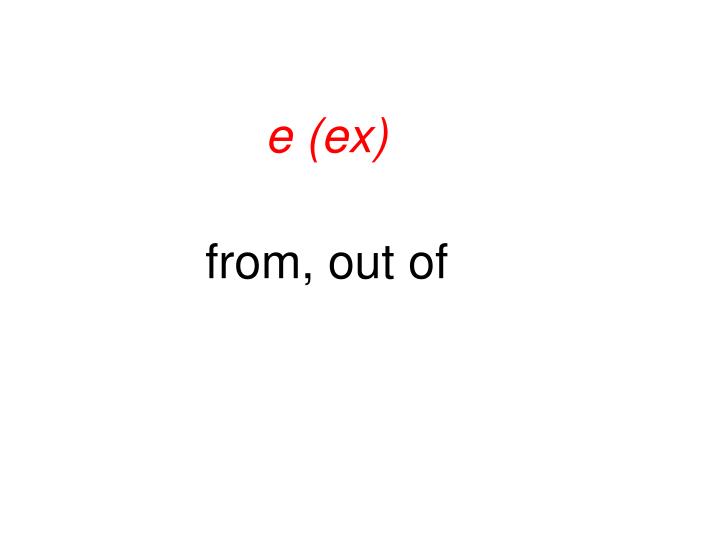The image features a very plain, predominantly white background with a minimalistic, centered text layout. At the top, in large, italicized, red lowercase font, is the letter "e," followed by red parentheses containing the italicized lowercase letters "x." Below this, separated by ample white space, the black text "from, out of" is presented in all lowercase letters. The red text uses a sans serif font, while the black definition text underneath shares the same sans serif style. The overall composition, using only the colors red and black, suggests a simplified dictionary-like definition of "ex."